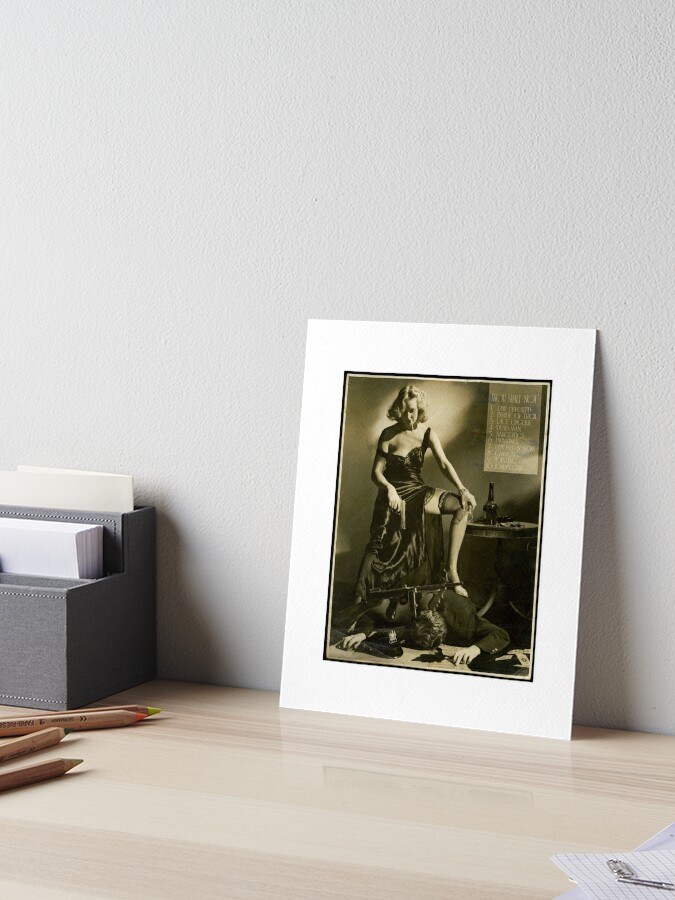The image depicts an indoor setting with artificial lighting, showcasing the top of a light-stained wooden desk against a light gray wall. Leaning against the wall is a vertically rectangular, sepia-filtered picture frame. The picture within the frame features a dramatic scene: a woman in a dress, with one strap off her shoulder and her left leg placed dominantly on the back of a man lying face down on the ground. She holds a pistol in her right hand, aimed at the man, who has a notable Tommy gun on his back and apparent blood around him. The desk is adorned with several items including a bunch of colored wooden pencils (notably yellow, orange, and regular-colored) on the left side, a gray box containing white cards or sheets of paper, and a pad of paper with a couple of paperclips in the lower right corner. Additionally, there appears to be a bottle, possibly wine, placed on the table, contributing to the detailed setting of the room.